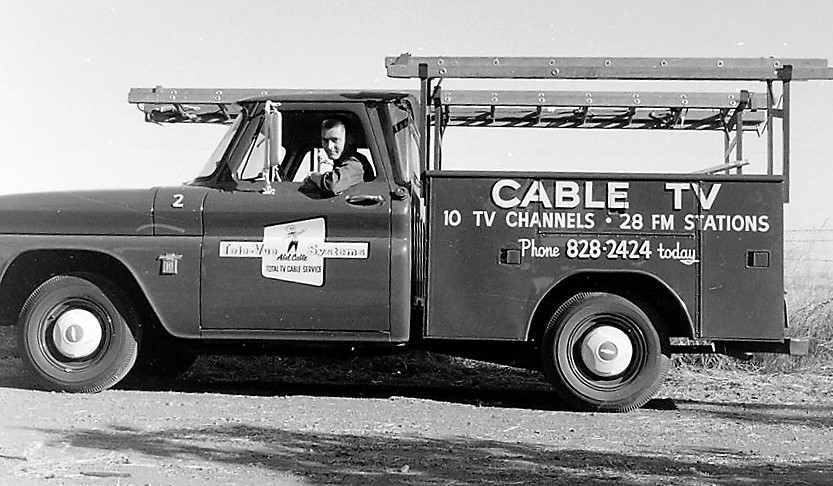This black and white, horizontal photograph captures an old utility truck parked outdoors on a dirt road, with an empty field and a white sky in the background. The truck, which appears dark in color, features prominent white text on its side advertising "Cable TV, 10 TV channels, 28 FM stations" and provides a contact number "phone 828-2424." The vehicle, possibly used for installations or repairs, includes two ladders mounted on its rear bed and displays a difficult-to-read logo related to cable TV services on the driver’s door. In the driver's seat, a Caucasian man with pale skin and wearing a dark-colored long-sleeve shirt gazes out confidently toward the camera, his elbow resting casually on the window ledge. The truck's black tires and likely silver hubcaps add to the classic utility vehicle's appearance.